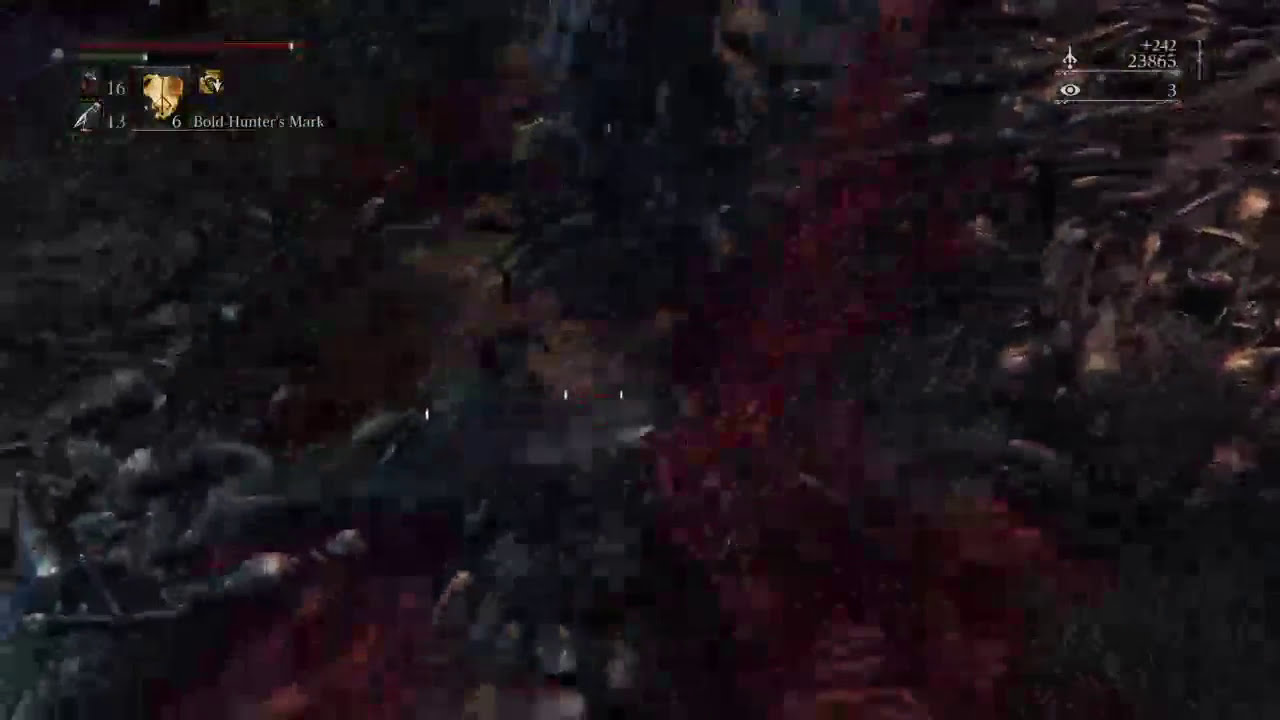The image is a blurry and dark screenshot from a video game, showcasing a battlefield scene with various game interface elements. In the upper left corner, the text "Bold Hunter's Mark" is displayed alongside three numbers: 16, 13, and 6, each next to its own emblem. Below these numbers, there are green and red status bars, which might represent health or experience. The left side of the image is primarily gray, transitioning to brown land in the middle, and a vivid red area that runs from top to bottom on the right. The far right of the image features what appear to be buildings. In the upper right corner, there's a spaceship icon with the numbers +242 and 23865 beneath it, and an eye icon with a "3" next to it. The overall scene includes gray, warrior-like figures engaging in combat, with red possibly indicating blood. The action seems chaotic, with points being added as characters are attacked and killed. The pixelated quality makes it difficult to discern finer details, but the contrasting colors and interface elements suggest a dynamic and intense gameplay environment.